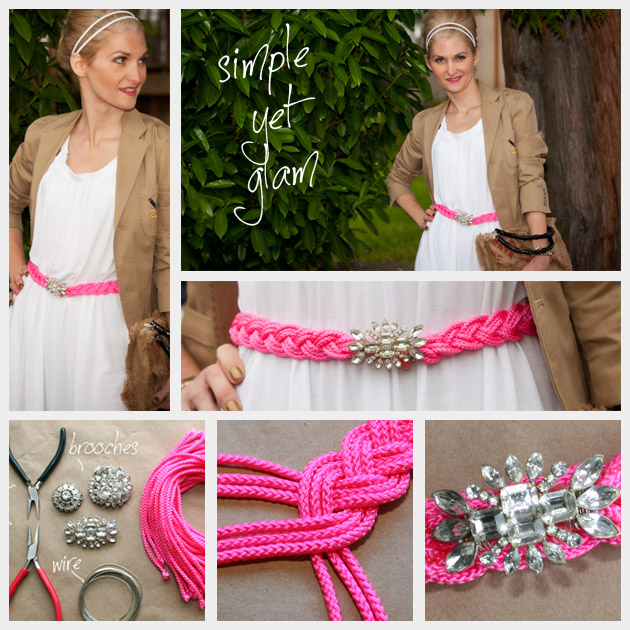The advertisement features a meticulously arranged collage showcasing a fashionable ensemble with the tagline "Simple Yet Glam." At the forefront, a blonde, middle-aged woman dons a stylish outfit composed of a white dress paired with a light tan blazer, accessorized with a headband delicately holding back her hair. She showcases a striking hot pink, rope-style belt adorned with an ornate diamond brooch prominently at her waist.

The image to the top left highlights the full outfit, emphasizing the belt's unique texture and the sophisticated contrast of her blazer. Adjacent to this, the central image magnifies the distinctive pink woven belt, drawing attention to the intricate brooch detail. Below, smaller inset images delve deeper into the features of the accessories, displaying additional brooch options and offering a closer look at the belt's craftsmanship.

To the upper right, the same model is portrayed holding a dark brown handbag, presumably with a rope-like handle, adding to the ensemble's cohesive elegance. The array of images at the bottom, including the tools and materials involved, underscores the handcrafted nature of the accessories being promoted. The entire composition aligns to exhibit finely curated, handcrafted belts and jewelry, epitomizing the 'simple yet glam' aesthetic.